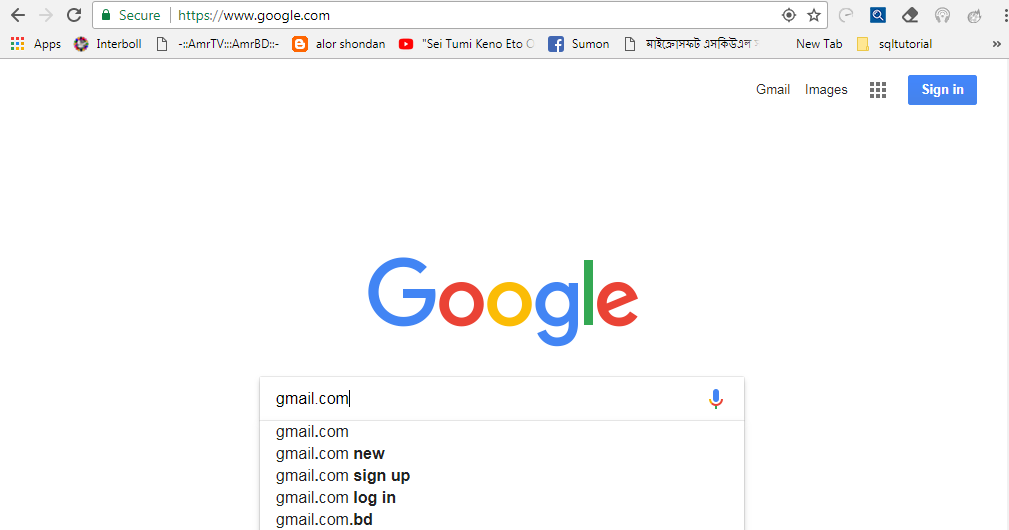Here is a detailed and cleaned-up caption for the image described:

---

This image captures a Google search page. At the top, there is a gray navigation bar featuring the back, forward, and refresh buttons, followed by the search bar, which displays the URL: "https://www.google.com". Below the navigation bar, several shortcut icons and text elements are arranged, including apps like Interval, AMRTV, Alor, and Shondan, along with buttons for YouTube and Facebook. Some text appears to be in Sanskrit. 

The main section of the Google page is shown beneath these shortcuts. On the upper right corner, black text links for "Gmail" and "Images" are present, next to a blue "Sign in" button. Central to the page is the iconic, large, multicolored Google logo. Below the logo is an expanded search bar with a prompt showing "gmail.com". This bar displays autocomplete suggestions such as “gmail.com,” “gmail.com new,” “gmail.com sign up,” “gmail.com log in,” and “gmail.com.bd”. A colored microphone icon is located on the right side of the search bar, indicating voice search functionality. 

Overall, this capture showcases the typical elements of a Google search page interface.